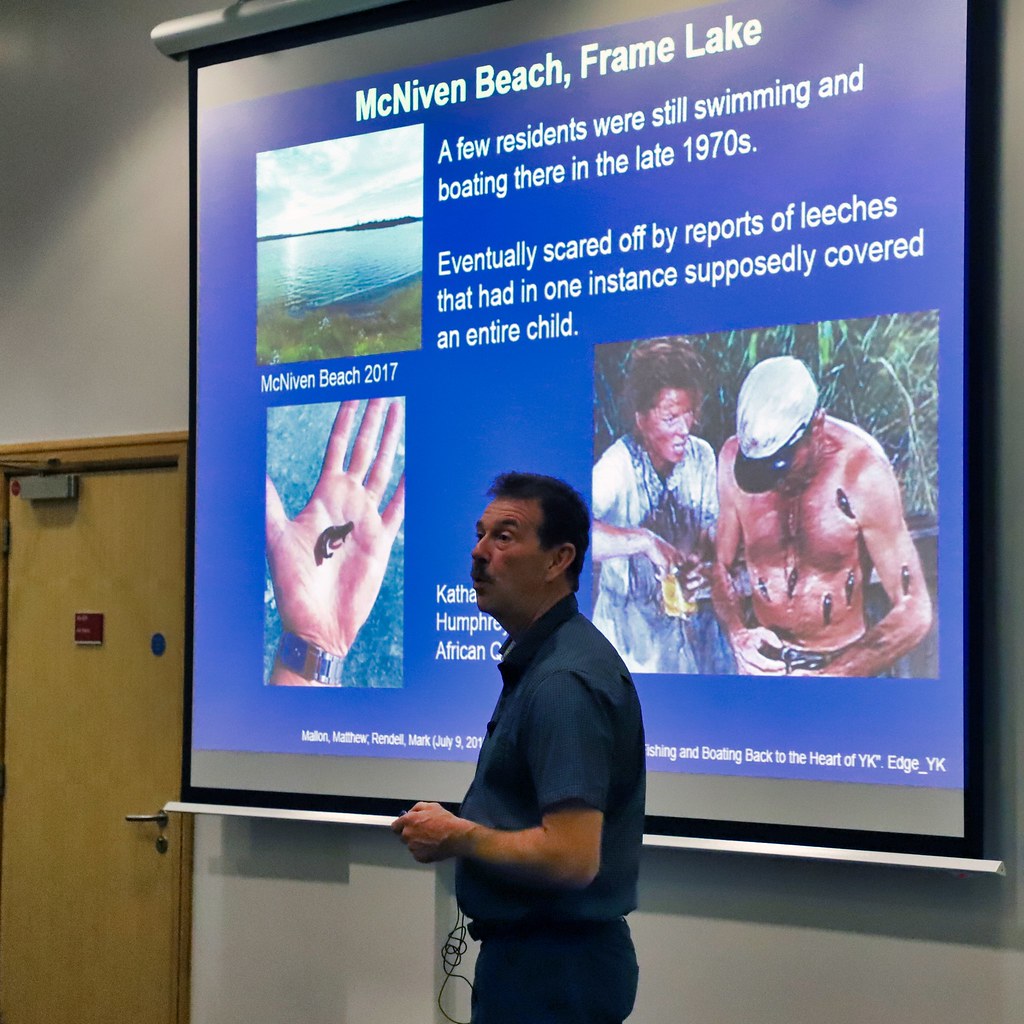The square-format color photograph depicts a man, likely a teacher or professor, standing slightly to the side, presenting to an unseen audience. He is attired in a blue collared shirt and black pants, and sports dark hair and a mustache. Behind him is a white wall with dimmed overhead lighting that casts a spotlight on a large drop-down projection screen. This screen features a slide with a bright blue background, entitled "McNiven Beach, Frame Lake." The slide includes three images: at the top left, a photo labeled "McNiven Beach 2017" shows a sunny lake shoreline; below it, a picture of a hand holding a leech; and to the right, an illustration of a shirtless man covered in leeches while a woman attempts to remove them. The accompanying text reads: "A few residents were still swimming and boating there in the late 1970s, eventually scared off by reports of leeches that had in one instance supposedly covered an entire child." To the left of the screen is a solid, tan wood grain door with a self-closing mechanism and a silver push-down handle, adorned with a red sign likely indicating building directions. The entire setting suggests an educational environment such as a classroom or seminar.